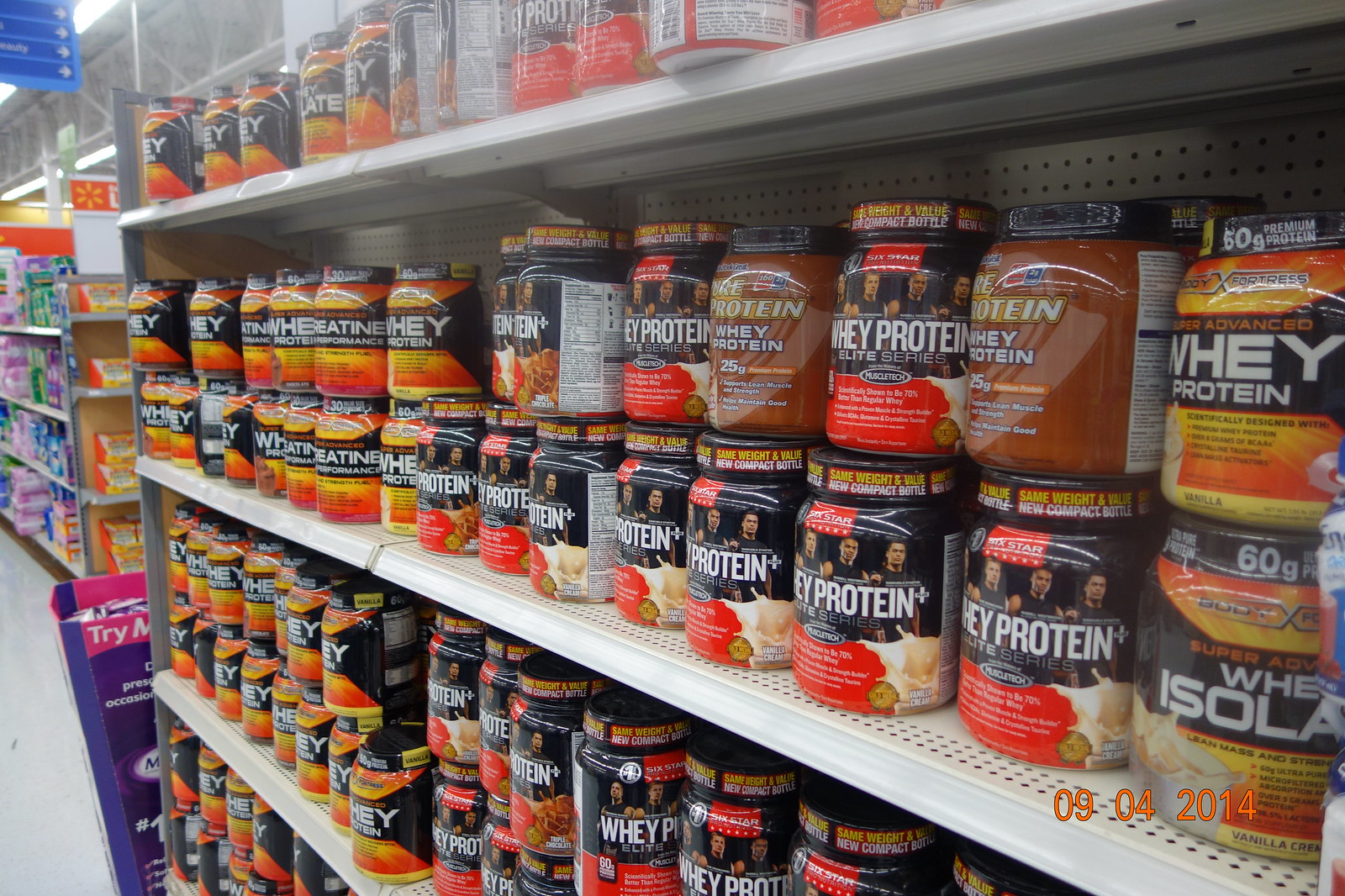The image showcases a vibrant vitamin and supplement store. The shelves, predominantly white, are stocked with a diverse array of protein jars in various colors, including red and orange. Near the top left corner, dark blue rectangles and arrows point to the right, possibly guiding visitors or indicating sections. Metal railings crown the upper part of the shelves. The store’s walls are painted a warm orange, complementing the bright, clean, white floor. 

One jar prominently features an orange design with a yellow burst in the center, emblazoned with the text "We Isolate" or "Whey Isolate." Additionally, vivid graphics, including splashes of liquid on some jars, enhance the aesthetic appeal of the display. The scene also includes posters or images of three professional fighters endorsing the products. Noticeable among the variety are jars labeled as creatine and other specialized supplements, catering to fitness enthusiasts and athletes aiming for peak performance.